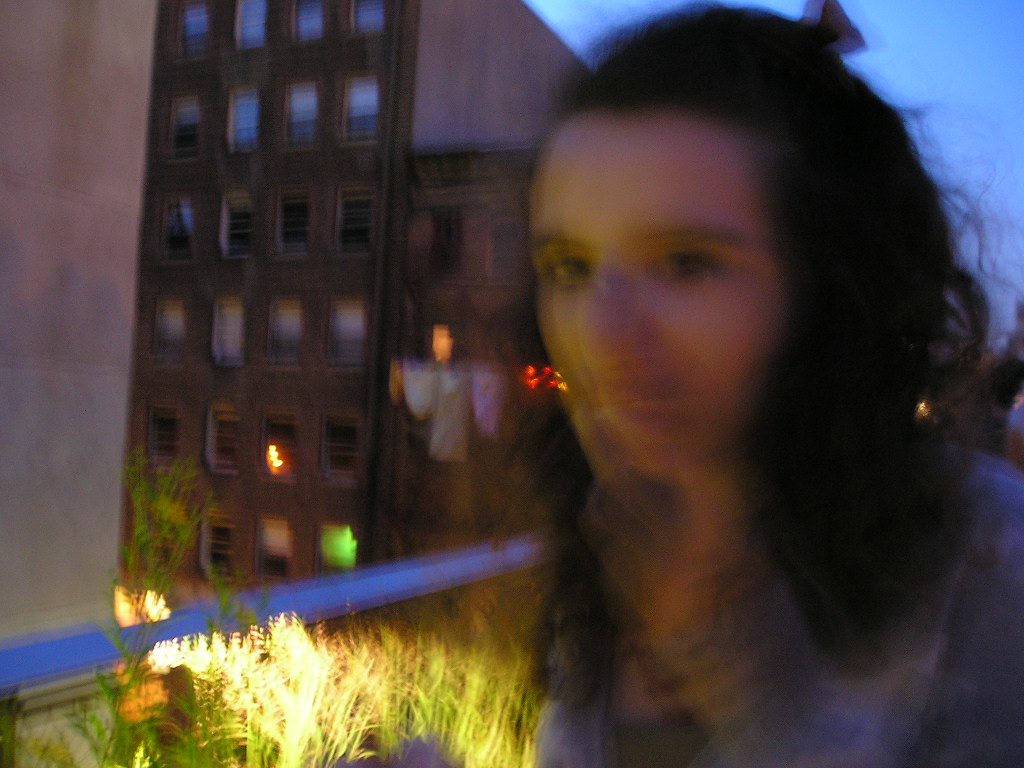In this blurred photo, a young woman, likely in her 20s, stands on an illuminated patio amidst an urban setting characterized by tall buildings. The patio is adorned with light-wrapped plants that add a gentle glow to the scene. Although details of her face are indistinct, her brown eyes and eyebrows are slightly discernible. She has short, curly hair and her hand is raised near her face, in motion, contributing to the blurriness. The twilight sky casts a blue hue over the scene, suggesting that the sun has just set, leaving a faint afterglow.